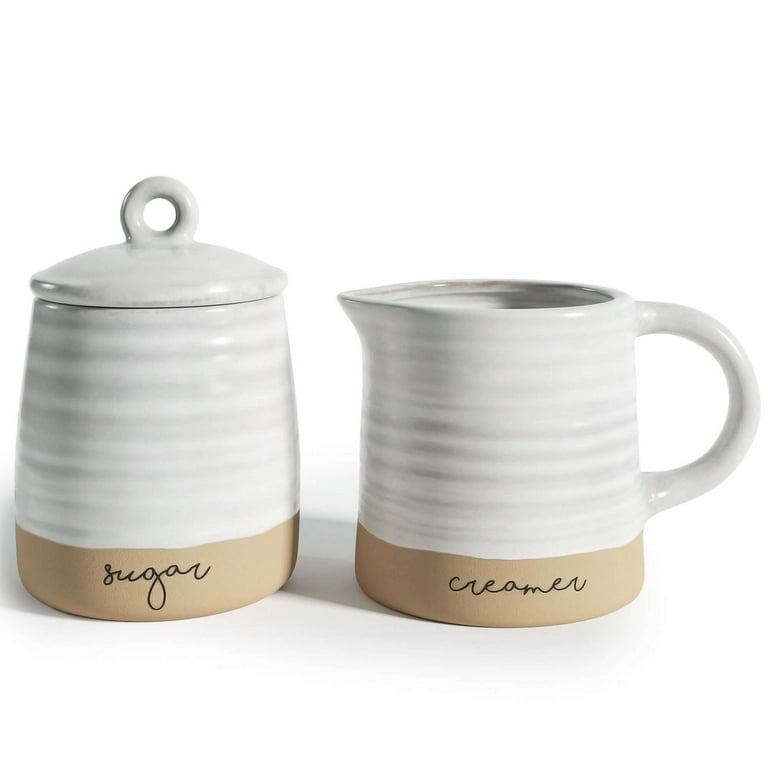The image showcases two handmade ceramic containers, both painted in a glossy white finish. These containers are adorned with a lighter tan border, approximately one inch tall, encircling their bottoms. The container on the left, which serves as a sugar cup, has "sugar" written in black cursive on its tan border and features a lid with a small circular hoop handle that includes a hole in the middle. The container on the right, intended for creamer, resembles a coffee mug with a handle facing the right side and a small spout on the left side of its rim. It also bears the word "creamer" in black cursive on its tan border. Both containers feature delicate circular line patterns and cast subtle shadows against the white background.